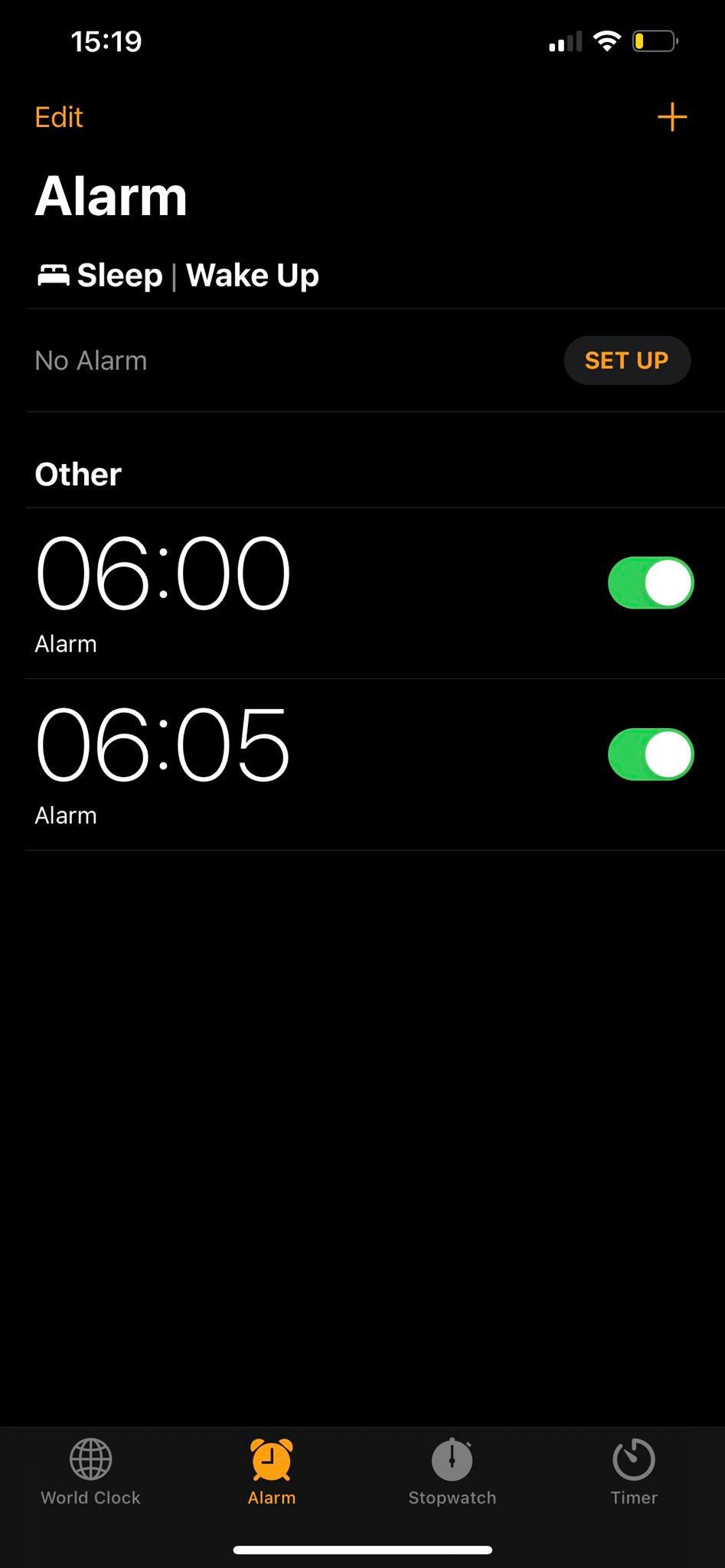The screen capture displays the alarm settings on a smartphone. The time is currently 15:19, and the phone shows a reception strength of two out of four bars. The battery is critically low at approximately 15%, but the device is connected to a strong Wi-Fi network. In the alarm settings menu, options for 'Sleep' and 'Wake Up' are visible with the current status set to 'No Alarm'. Additionally, there are two alarms configured: the first set for 6:00 AM and a backup shortly after at 6:05 AM, both indicated as active with their corresponding switches toggled on. At the bottom of the screen, the navigation options for 'World Clock,' 'Alarm' (highlighted), 'Stopwatch,' and 'Timer' are clearly displayed.